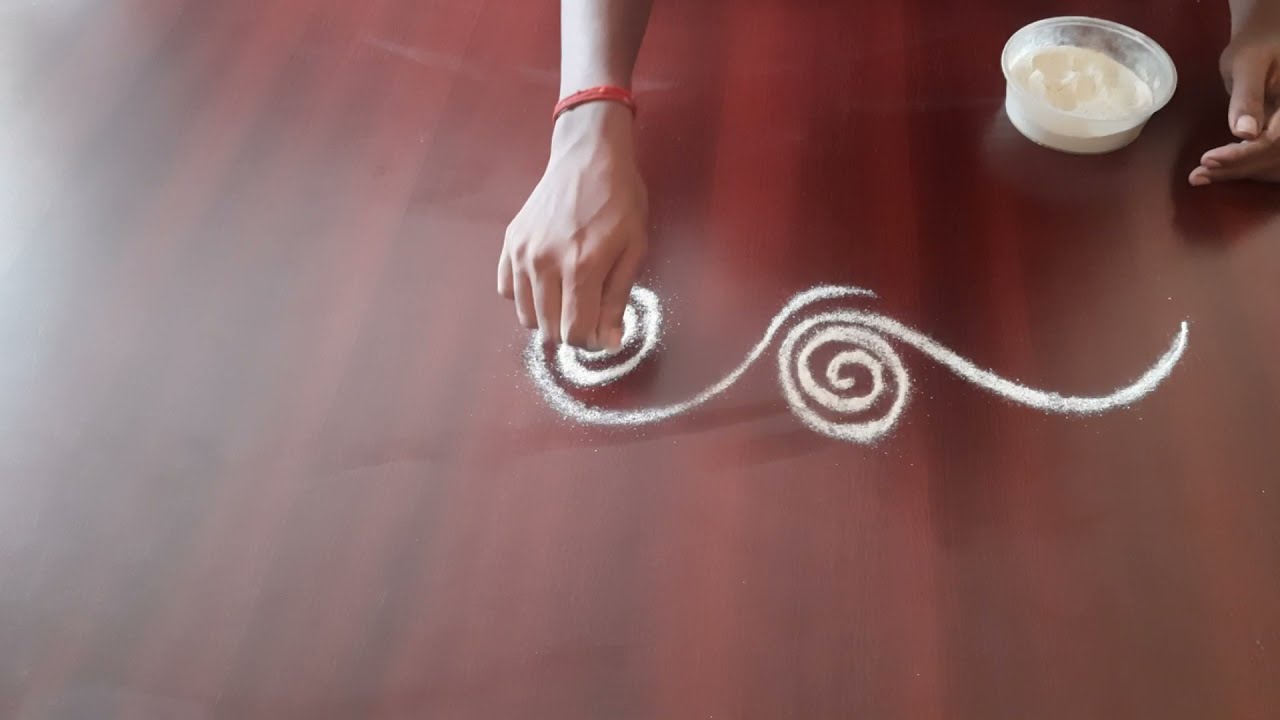The image captures a person meticulously creating spiral designs with a white powder on what appears to be a redwood surface, which could be either a table or the floor. The richly-hued, reflective redwood takes up most of the image, with two visible hands engaged in the artistic process. One hand, adorned with a tightly fitting rubber bracelet, emerges from the top of the frame, delicately distributing the powder into intricate, curlicue patterns. To the right lies a bowl or dish containing the white powder, which several observers have noted might be ground chalk or a similar material. The spirals, each looped twice with a long tail, are positioned close to each other. While the well-lit left side of the redwood surface enhances the contrast of the swirls, the light becomes less reflective on the right, drawing attention to the artist’s careful work in progress.